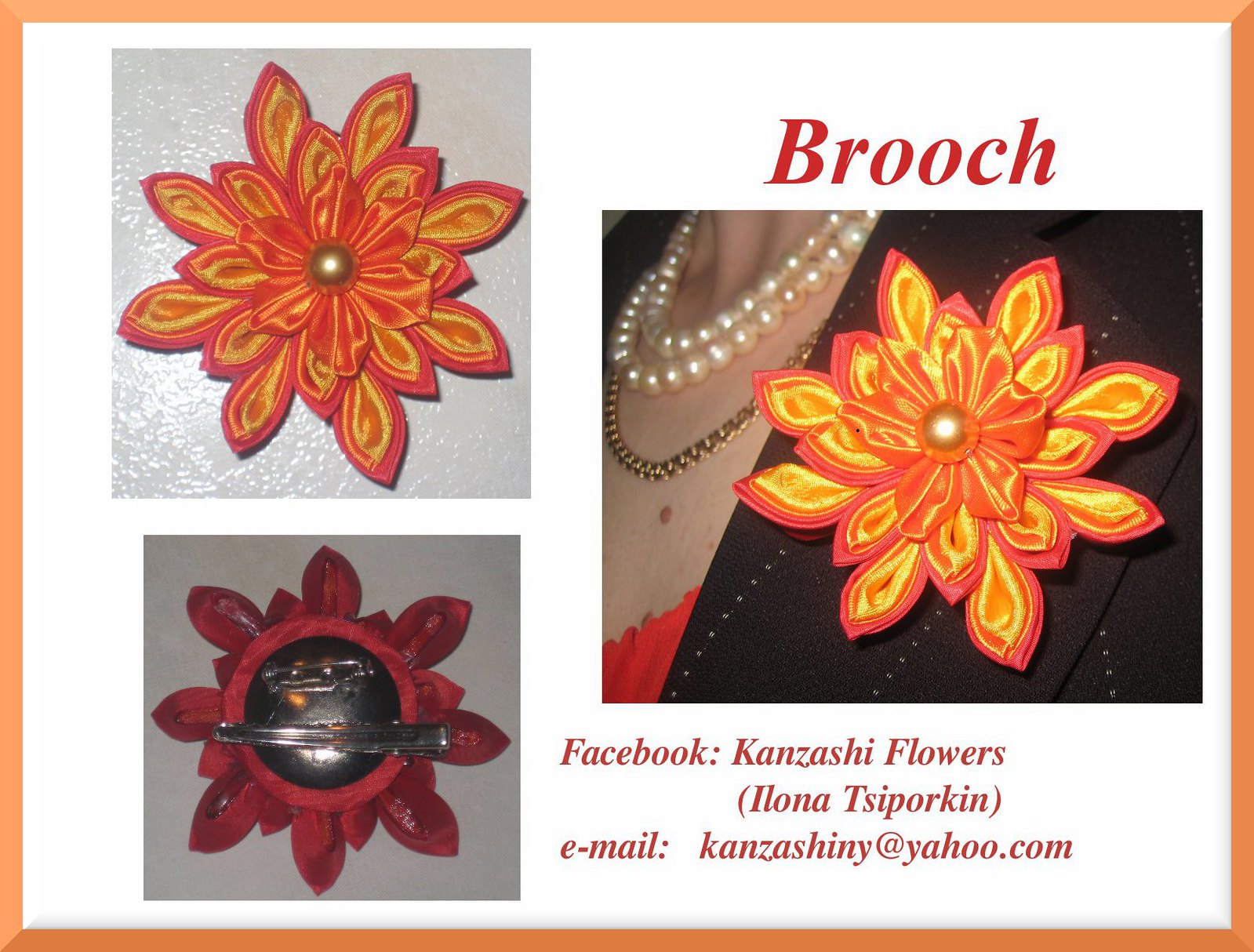The advertisement is a detailed, multi-image graphic promoting brooches by Ilona Tysborkan. The central visual is framed with an orange outline on a white background. A larger image of a brooch, featuring a pearl at its center and orange to dark reddish petals, is prominently displayed on the right side. This brooch has a silky texture and is pinned on the lapel of a black blazer worn over a red shirt. The woman wearing it is adorned with two pearl necklaces and a darker pearl necklace, and she has a notable mole on her chest. Above this larger brooch image, the word "Brooch" is written in bold red letters. On the left side of the advertisement, two smaller images: the top one mirrors the main brooch on a gray background, while the bottom one displays a red-style flower with a dark center. An image at the bottom left corner showcases the back of the brooch, revealing a silver pin or clip. Below the larger brooch image, it includes the text "Facebook, Kanzashi Flowers, Ilona Tysborkan" along with the email address "kanzashiny@yahoo.com."